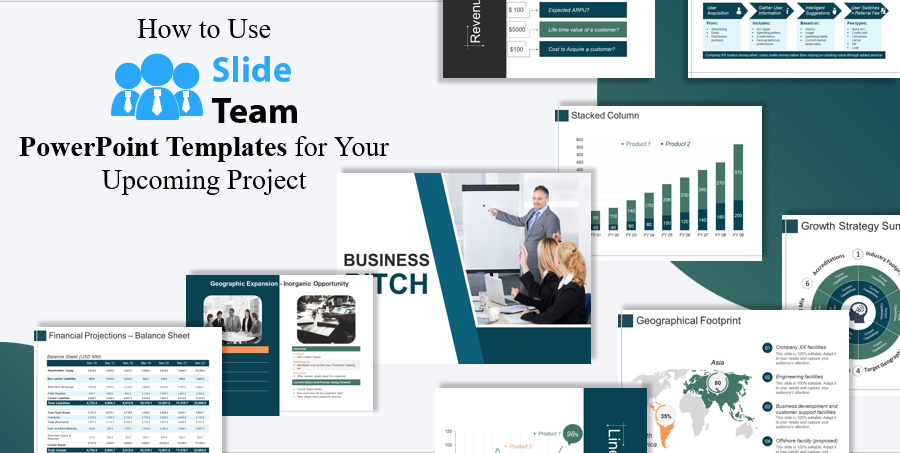The image is a wide, colorful graphic serving as a detailed cover, possibly for a YouTube video, on using Slide Team PowerPoint templates for business projects. Dominated by the title, "How to Use Slide Team PowerPoint Templates for Your Upcoming Project," the upper left corner features text along with a simple pictogram logo of three blue, tie-wearing figures symbolizing the slide team. The slide is dense with various smaller slides and infographics, showcasing diverse functionalities like graphs, tables for financial projections, maps, and bullet points. Among the visual elements, there are bar charts, both vertical and horizontal, a slide labeled "business TCH" (partly obscured), and a photo of a person presenting at a business meeting. Each screenshot is presented with a drop shadow, emphasizing the professional and multifaceted capability of the templates.